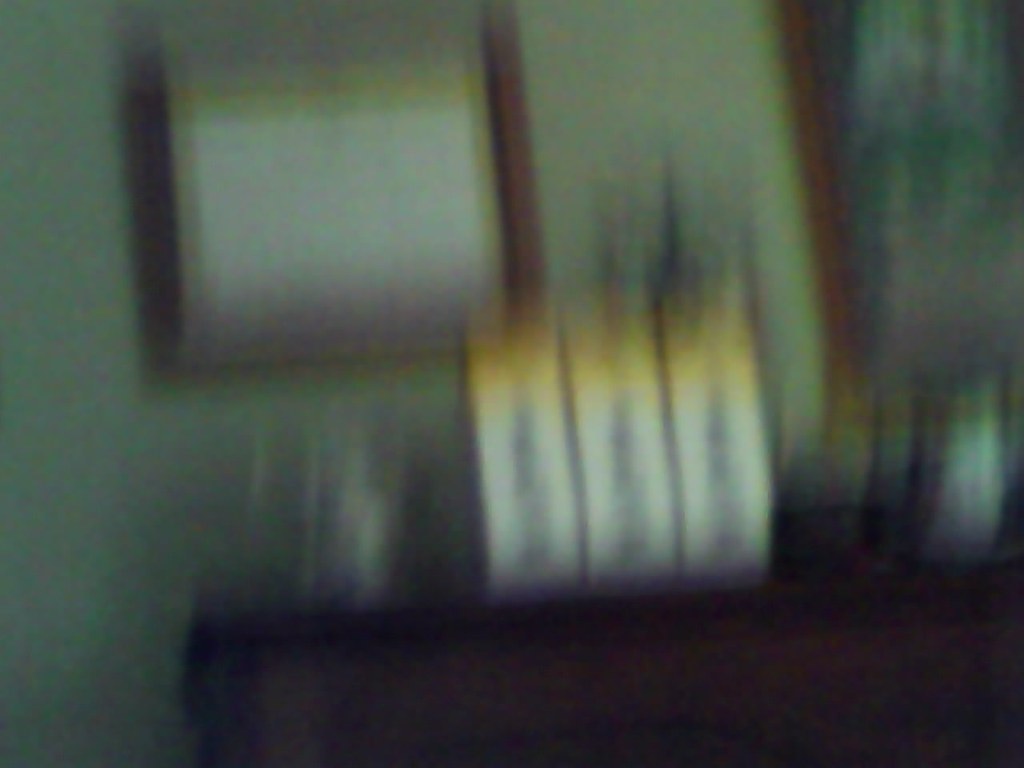This image is an extremely blurry photograph likely taken in what seems to be a hotel room, casting it in a hazy and unclear light. The snapshot, plagued by motion blur, perhaps from vertical camera movement, makes it difficult to perceive the exact details or nature of the objects in the room. The room's background features a wall that appears greenish-gray due to the lighting and blur. There might be a window or a bulletin board on this wall, next to what could be a door. 

In the foreground, there's a rectangular, black wooden structure, possibly a nightstand or mantelpiece, that spans most of the width of the image and is tilted slightly at about a 10-degree angle. On this structure, three long striped white lines, which turn yellow at their jagged tops, protrude upward. These could be misinterpreted as pieces of text or objects due to their blurry presentation. 

Additionally, there seems to be a calendar with a yellow border on the wall, complemented by a vague impression of a painting resembling a Monet, framed in brown wood, with hints of greens and blues adding to the room's possibly artistic ambiance. The combined vague shapes and colors create a confusing yet intriguing visual narrative, leaving much to the imagination.